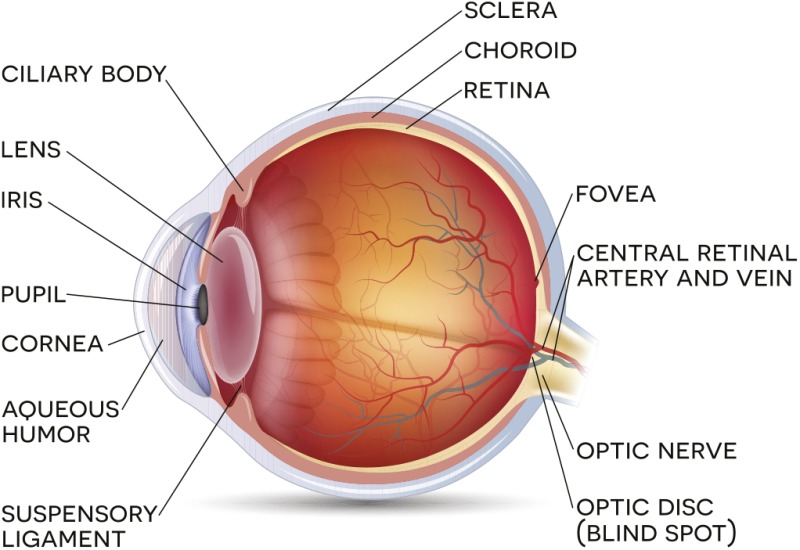This is a detailed, labeled illustration of the human eye on a white background, presented as a side view. The image meticulously identifies various parts of the eye, with black text labels and lines pointing to specific areas. Key components labeled include the ciliary body, lens, iris, pupil, cornea, aqueous humor, suspensory ligament, optic disc (also known as the blind spot), optic nerve, central retinal artery and vein, fovea, retina, choroid, and sclera. The inner part of the eye is shown in red with small veins, highlighting the central retinal artery and vein as well as the optic nerve. Layers of the eye are depicted progressively from the innermost retina to the outer choroid and sclera. The illustration also details the differentiation of the black regions of the iris and pupil, while the pink area signifies the lens.